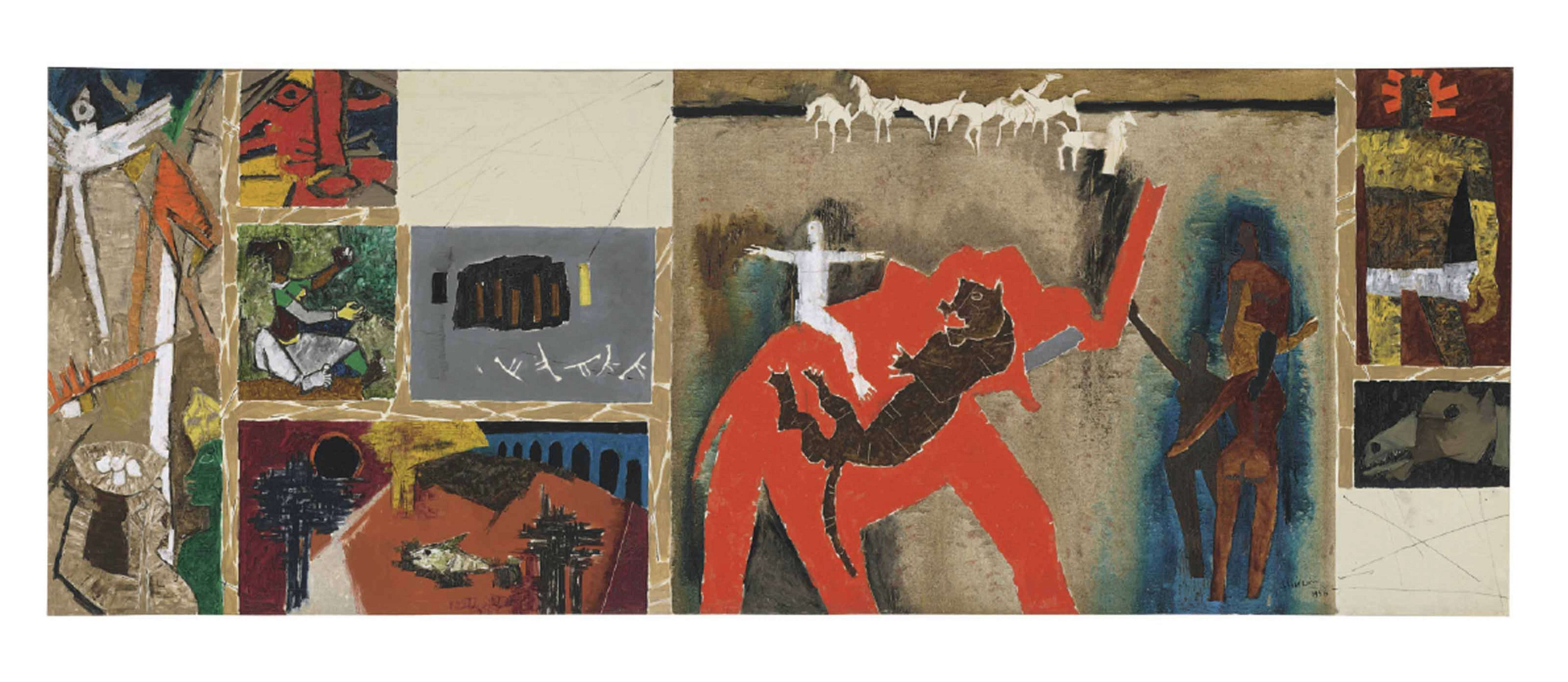The artwork is an expansive, widescreen abstract painting, reminiscent of cave or wall drawings, with a variety of vivid and intricate details. Dominated by a mosaic of squares, each housing its own unique illustration, the focal point is a large, eye-catching square containing a surreal mélange: tiny white horses galloping at the top and a strikingly red elephant carrying a white-figured man on its back. Adding to the surrealism, an upside-down cat appears to rest upon the red elephant's surface. To the right of this central scene, there are nude figures positioned next to a man with red lines emanating from his head, set against gold and white hues.

On the left side, various individual drawings populate a grayish-white background. Among these, a dark-skinned woman sits serenely in a dress, a dark-skinned girl sits on the ground, and a boy appears engaged in creating art on a large table. Above these figures, a brown-haired angel with white wings is depicted alongside a bird bath. Additional elements include a fish laid out on a table at the bottom and abstract brown logs. The middle section of the painting includes an animal resembling a panther sitting atop the red elephant.

Colors blend seamlessly throughout the entire piece with shades of white, tan, orange, burgundy, blue, gold, and gray, creating an intricate tapestry that defies simple interpretation. The rightmost section features a diverse array of smaller scenes, including another person with brown hair and additional abstract, yellow and brown-toned paintings. The overall effect is a unique and mesmerizing puzzle that invites viewers to explore its multiplicity of forms and colors.